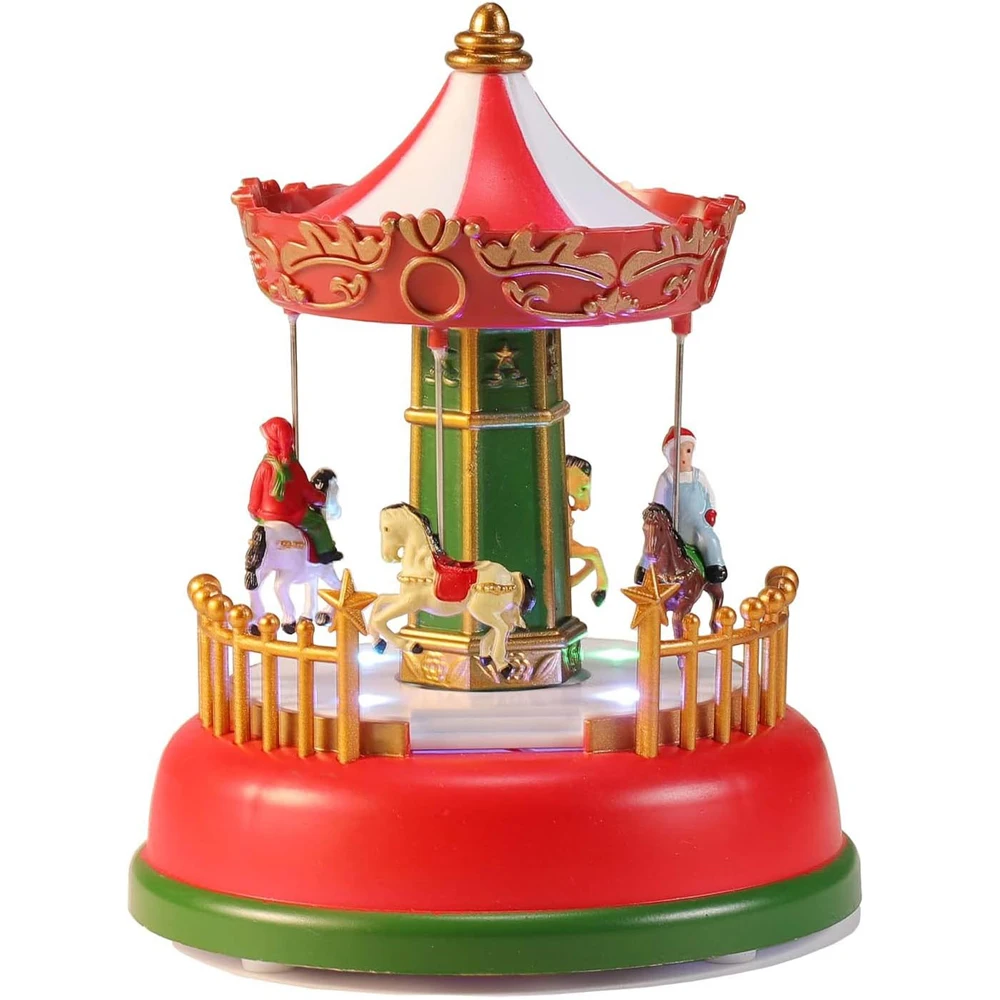This is a detailed photo of an old toy carousel, meticulously crafted to evoke the charm of a classic merry-go-round. The base of the carousel is a light green color, supporting a layer of red above it, and this foundation is encircled by a delicate gold fence. At the center of the carousel stands a green and gold centerpiece, crowned by a striking red and white striped canopy with a red border adorned with gold leaves and engravings, culminating in a gold ornament at the top. There are four horses on this carousel, each mounted on silver poles. Two of these horses carry tiny riders: one wearing blue overalls, a white shirt, a red hat, and red gloves, facing the camera; and the other in a red jacket and green pants, facing away. These details breathe life into the whimsical scene, capturing the nostalgic essence of an amusement park attraction. The background is a stark white, drawing uninterrupted focus to the intricate and colorful details of this enchanting toy.